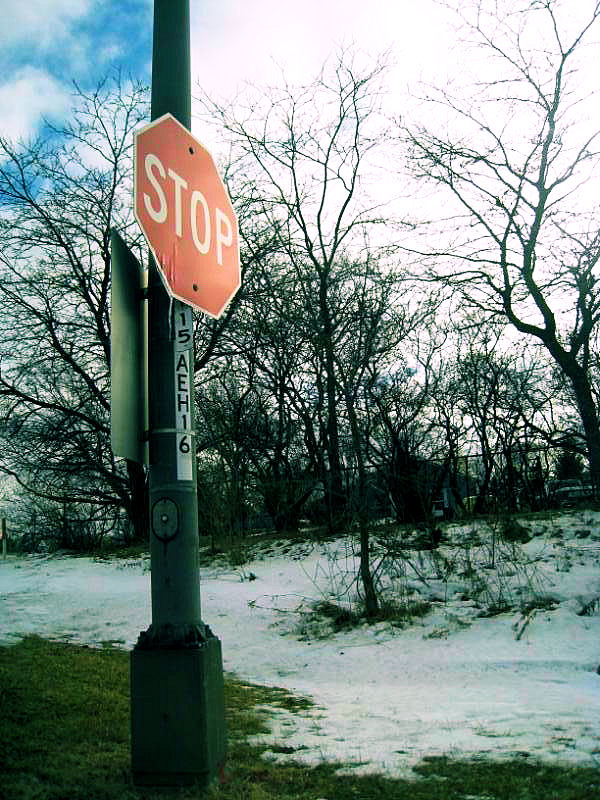The photograph depicts a wintry outdoor scene featuring a prominent stop sign attached to a metal pole, likely a light pole. The pole, positioned on the front left of the image, appears gray, though it's suggested it could be a dark green due to lighting conditions. Below the stop sign is a white sign with the code "15AEH16." The ground is lightly covered in snow, except for a small visible patch of green grass near the front. The terrain appears to be slightly uphill with more snow towards the back. Surrounding the area are leafless trees, indicating it's wintertime. In the background, there's a chain-link fence and potentially some obscured homes. The sky is predominantly cloudy with a hint of blue, suggesting that a snowstorm may have recently passed.